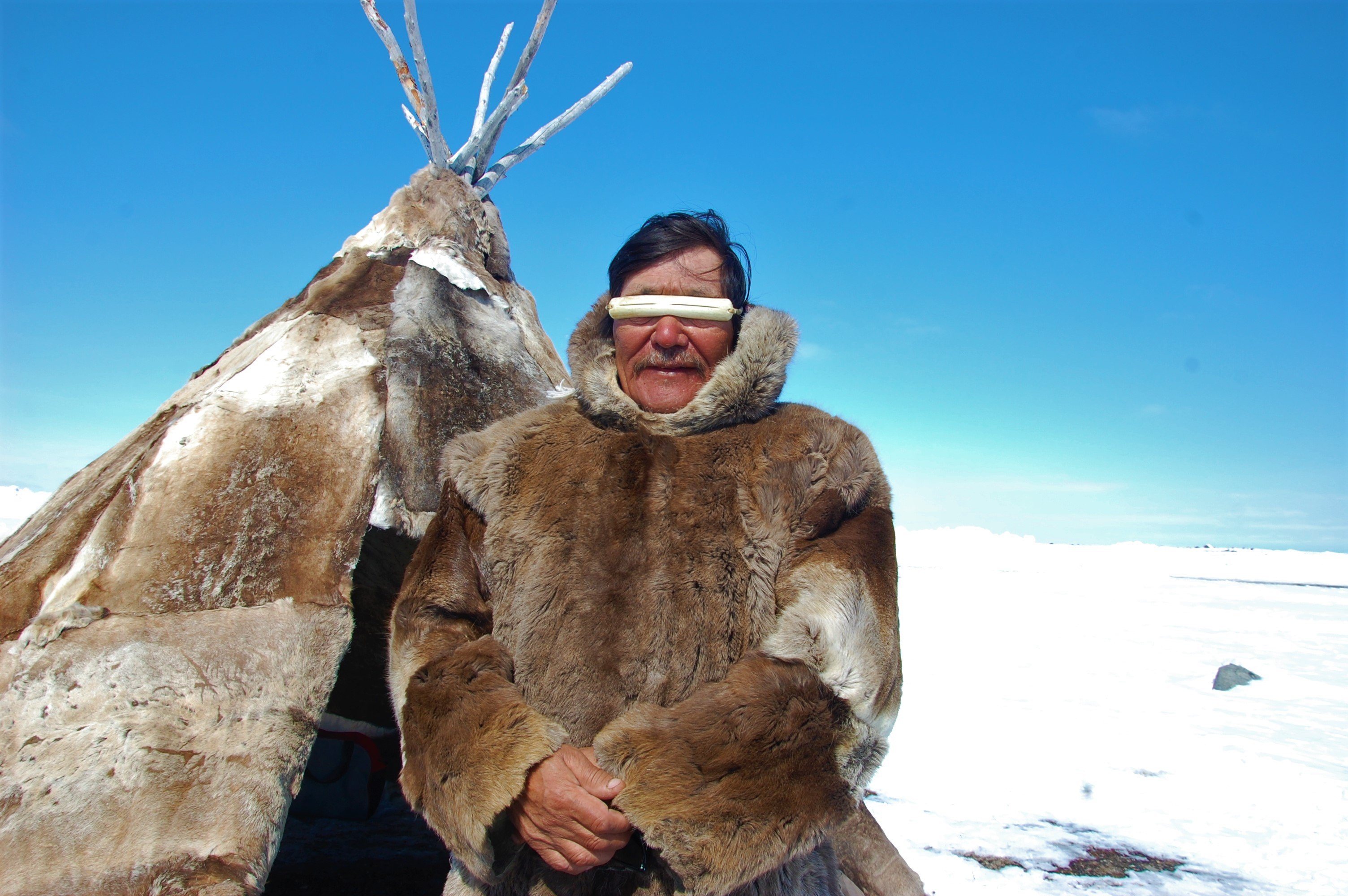This is a color photograph showcasing a man standing beside a teepee on a snow-covered landscape under a bright, clear blue sky. The teepee, situated in the foreground on the left, is adorned with animal hides in shades of light brown, gray, and white, with white sticks protruding from its top. The man stands near the teepee's opening, posed facing the camera with his hands clasped in front of him. He is dressed in a heavy fur coat made from various pieces of animal hide in brown and white, which extends down to his wrists and features a fuzzy hood that also warms his ears. Over his eyes, he wears distinctive white glasses, possibly made from a bleached material, adding a notable feature to his rugged attire. The image emanates a serene yet chilly atmosphere accentuated by the brilliant sunlight and vast expanse of white snow.